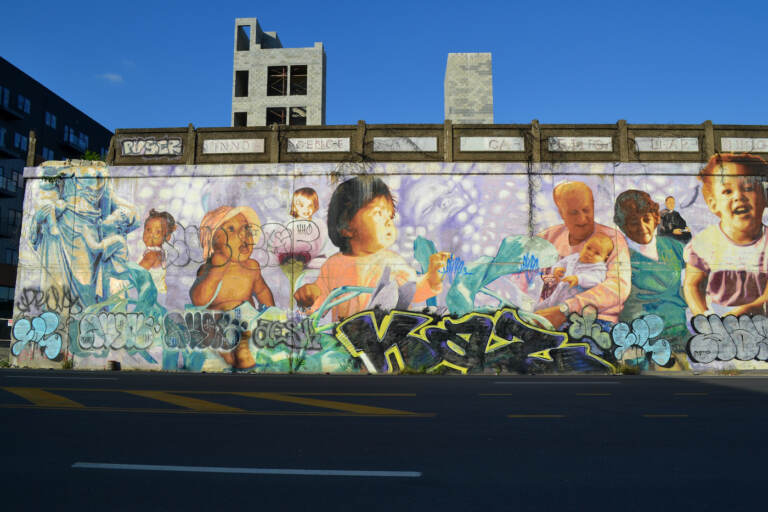The square, full-color photograph captures an outdoor scene on a clear day. The upper portion of the image showcases a bright blue sky without any clouds, with several gray buildings rising into view. On the far left, a darker building with numerous windows can be seen. The bottom of the image features a stretch of pavement marked by a white lane dividing line and yellow "stay out" lines. Dominating the scene is a large mural on the side of a wall, decorated with realistic images of people, primarily babies, with a couple of adults on the far right, one of whom is holding a baby. This mural is interspersed with various graffiti, including names and tags in black with yellow outlines, adding an additional layer of visual interest to the vibrant street artwork.